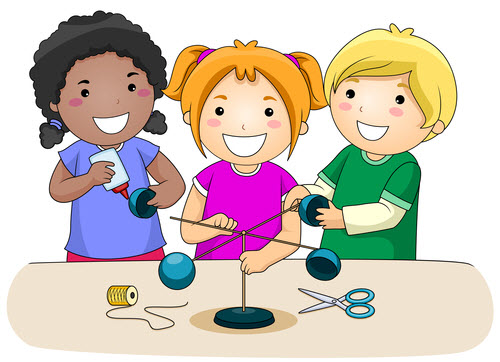This detailed image is a digital illustration or clipart of three cartoon toddlers—two girls and one boy—working on a science project. They are gathered around a light brown table, which has various crafting items scattered across it. In the center of the table, there is an object resembling a planetary system model. This model includes a thin stick anchored by a blue round base. At the top of the stick, two other sticks intersect to form a cross, with blue, illuminated spheres attached to each end. 

The girl on the left, who appears to be African American, has black pigtails, a darker skin tone, and is wearing a purple shirt, seemingly applying glue to one of the spheres. In the center is a girl with Caucasian features, orange hair in pigtails, and a bright pink shirt. She is handling another part of the model. The boy on the right, also Caucasian, has short blonde hair and is wearing a green shirt with a tan undershirt. He seems focused on affixing the blue spheres to the ends of the intersecting sticks.

Additional items on the table include a row of yellow thread on the left side and a pair of scissors with blue round handles on the right. The overall scene portrays a lively and collaborative effort among the kids as they construct their intricate and brightly colored science project.